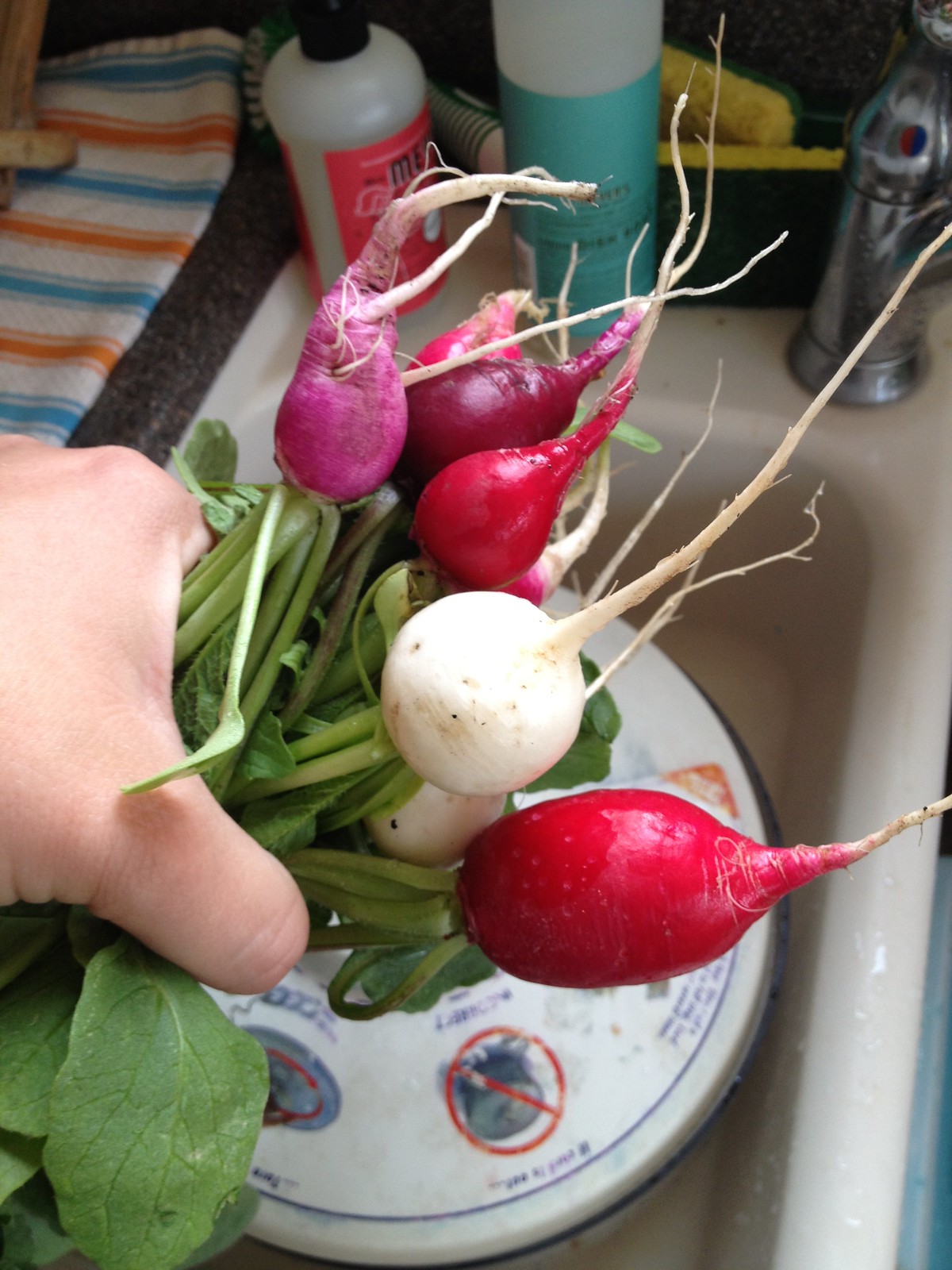The image is a portrait-mode photograph showcasing a Caucasian hand holding freshly uprooted root vegetables, predominantly beets, over a small, cream-colored ceramic sink. The vegetables, which include red, white, and purple beets, exhibit a shiny, freshly washed appearance with droplets of water. The beets are held by their leafy stalks, which are light and dark green and feature wavy edges with dark green ribs. Some of the vegetables show long, creamy sprouts at their tips.

In the background, the sink area is cluttered with details, including a white towel with light blue and red stripes in the top left corner and two Mrs. Meyers soap bottles—one with a red label and black cap, and the other with an aqua label—positioned on the ceramic sink frame. A yellow sponge with green trim and a silver faucet equipped with a red and blue temperature indicator are visible in the top right corner. The faucet spout is not visible, suggesting it is turned towards the other side of the sink. Beneath the vegetables, there is a stack of dishes, including a plate with a white, circular container that features red circles and other indeterminate images or patterns.